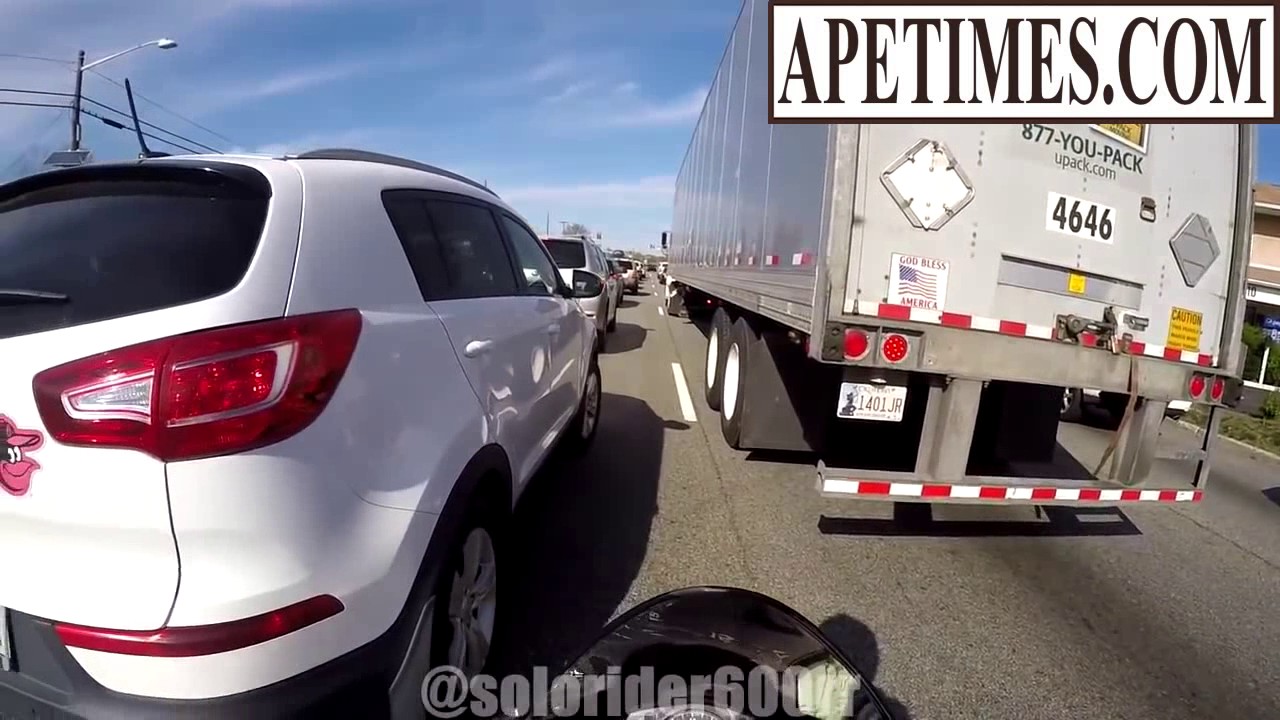In this busy freeway scene captured from a first-person perspective, likely that of a motorcycle rider, we see bumper-to-bumper traffic during what appears to be rush hour. The road is textured and worn with a white dotted paint line running down the middle. To the left is a white SUV proudly displaying a Baltimore Orioles sticker on its back, with glowing red taillights. On the right, a large silver and gray semi-truck dominates the view, bearing the phone number 877-U-PACK and the website address upack.com, as well as the number 4646. The truck is equipped with four reflectors, red and white checkered warning stripes, a caution sign, and other safety markings. In the bottom center of the image, the front end of a black motorcycle is visible, marked with a transparent white caption reading @SoloRider600. At the top right corner, the logo ApeTimes.com is prominently displayed. The photograph is set against a clear blue sky with scattered clouds, and hints of a residential building peek from behind the large trailer. Telephone poles with street lamps line the side, adding to the urban landscape of this congested highway scene.